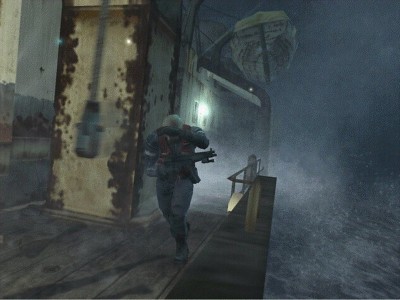This image is a screenshot from a video game likely from the late 90s to mid-2000s, displaying a character on a boat in turbulent weather. The sky is a dark, ominous mix of blue and gray, with lifting white fog adding to the ominous atmosphere. The water is a similarly dark blue with gray splotches, creating an impression of rough seas. The boat itself is a blend of chocolate brown and dark gray, rocking slightly due to the waves. The deck is partially obscured by shadows.

In the center, a character dressed in dark blue pants, a dark blue shirt, and a red vest is running towards the viewer at an angle. They are hastily covering their face with their right arm, and their left hand brandishes a gun pointed to the side. The character's salt-and-pepper hair stands out against the otherwise dark scene. 

The background is smoky and foggy, with blurry elements including a possible electronic device on the wall with something sticking out upwards. The overall scene is difficult to discern in detail due to the dark, foggy conditions, contributing to a foreboding, almost eerie atmosphere.